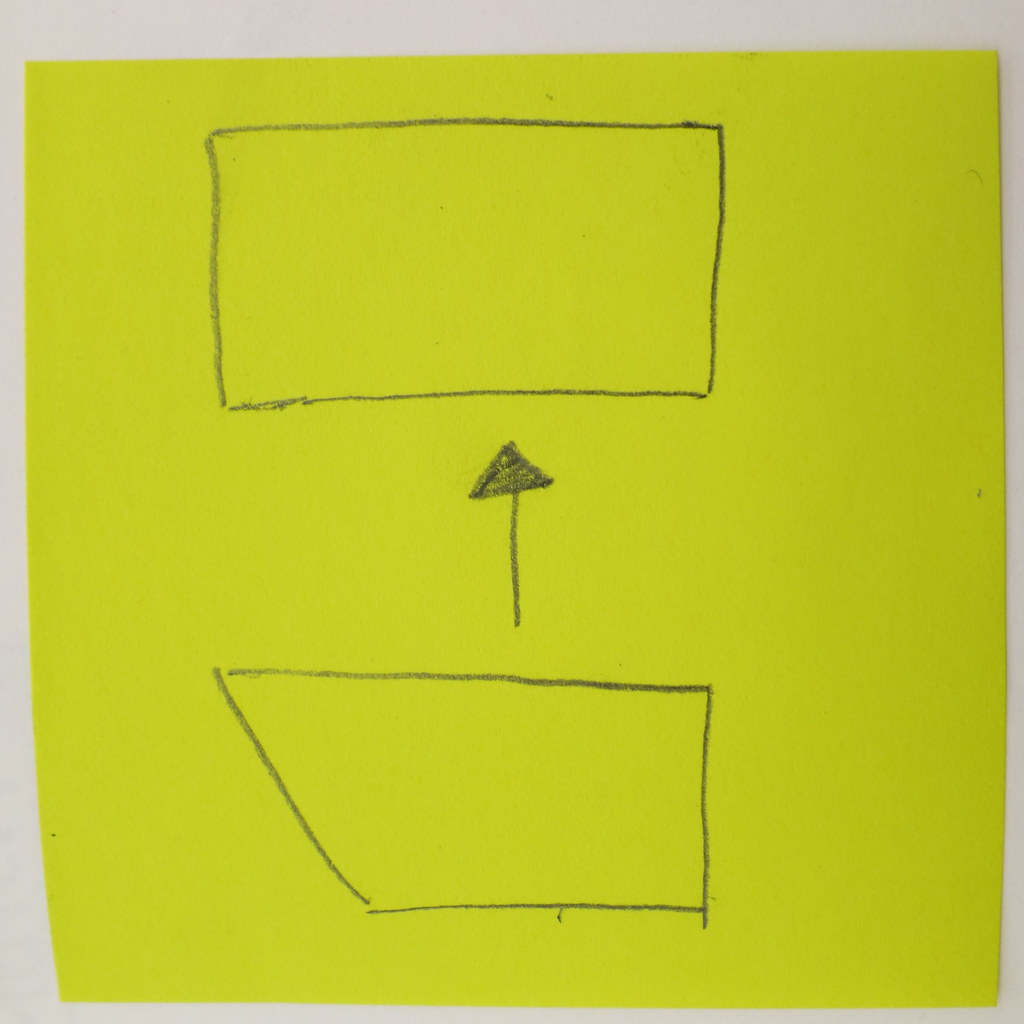A close-up photograph of a square lime green post-it note. The post-it note features three distinct elements drawn with what appears to be a dark graphite pencil. Centered in the top section is a hand-drawn rectangle, oriented horizontally with the width notably longer than the height. Near the bottom of the post-it note, there is a geometrically complex trapezoid, where the top side is longer and angled, creating a narrowing effect toward the bottom. The right-hand side of the trapezoid is vertical and straight, while the left-hand side slants inward from top to bottom. Positioned between these two shapes is an upward-pointing arrow. The arrow has a single straight line forming its shaft and a solid filled-in triangular head.